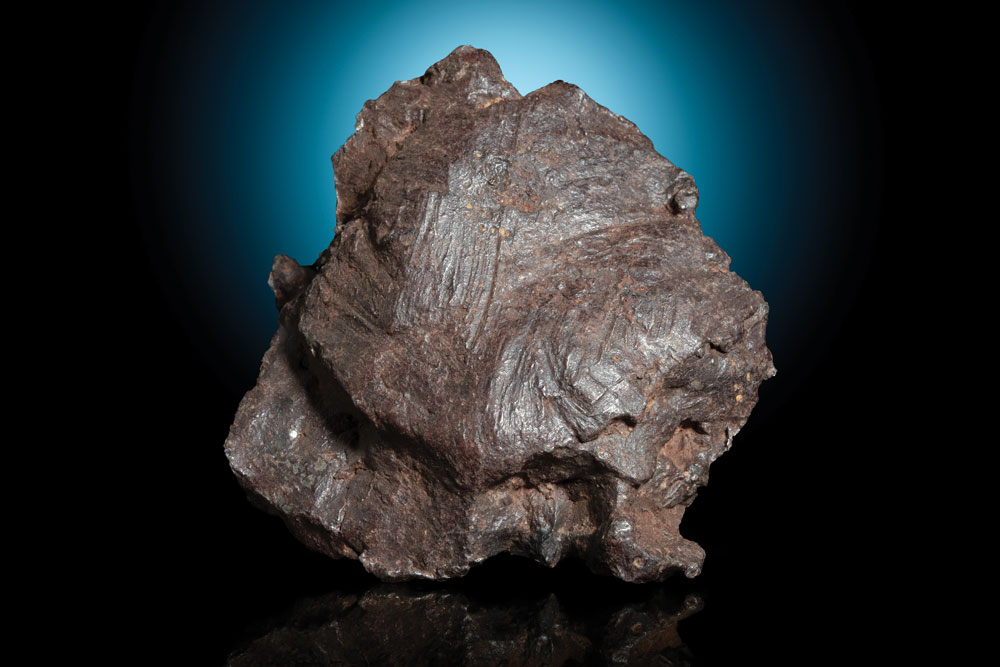This professionally shot photograph showcases a sizeable rock or statue, centrally displayed against a backdrop of a blue light that illuminates the middle, transitioning to a dark, almost black hue towards the edges. The foreground features a glossy black surface that reflects the rock, adding depth to the image. The rock itself is predominantly dark brown with a shiny, slightly coppery sheen, interspersed with flecks of lighter brown and possibly gray. Its jagged, unevenly circular shape gives it a mysterious, almost extraterrestrial appearance, leading to speculation that it might be a meteorite or a large, unrefined piece of ore, possibly copper. The intricate details of the rock, including its protrusions and grooves, suggest a blend of smooth and dull textures, enhancing its enigmatic charm. The absence of scale indicators makes it challenging to determine the rock's exact size, but its formidable presence implies significant weight and mass, fitting well in a museum or an academic display setup.